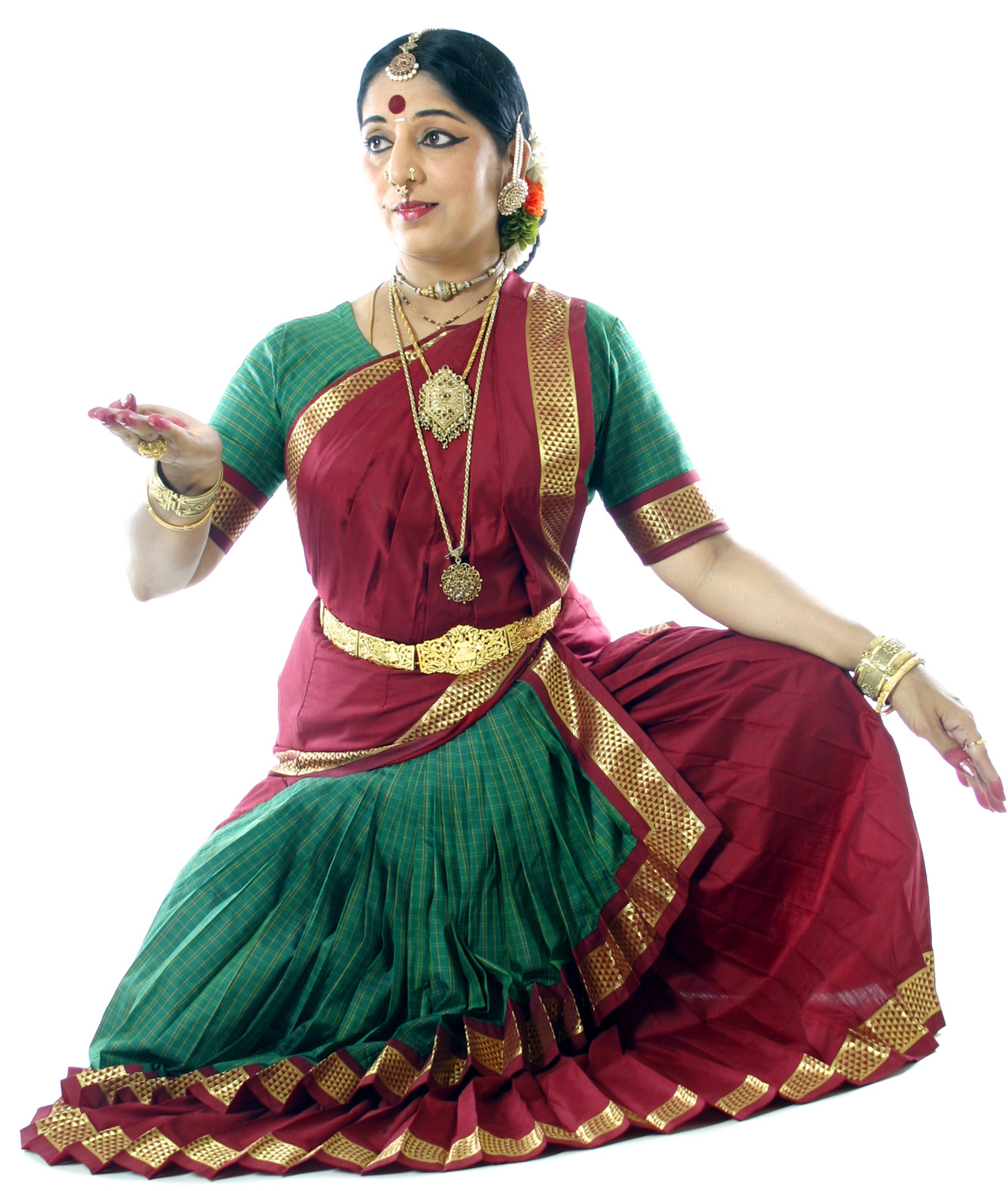This is a detailed image of a woman who appears to be Indian, dressed in traditional attire, possibly for a cultural celebration or ceremonial dance. She has brown hair adorned with jewelry at the parting and is distinguished by a red bindi on her forehead. Additionally, she sports a nose ring and prominent eyeliner accentuating her brown eyes. Her eyebrows match her hair color, and she is wearing red lipstick. 

Her outfit is a vibrant blend of green and red fabrics, intricately detailed with silver and gold accents. The dress features a silver belt and silver embellishments at the hem. Complementing her attire, she wears an array of gold jewelry, including gold earrings, heavy bracelets, and a set of three necklaces - a choker and two longer necklaces of varying lengths. 

Her hands are adorned with red nail polish, and she is posed gracefully on the ground. She is kneeling with one knee down and the other up, holding her right hand up in a traditional pose while her left hand rests on her knee. Her gaze is directed to her right, giving the impression of her being lost in thought or focusing on something in the distance. Her still and poised demeanor enhances the cultural and ceremonial essence of the image.